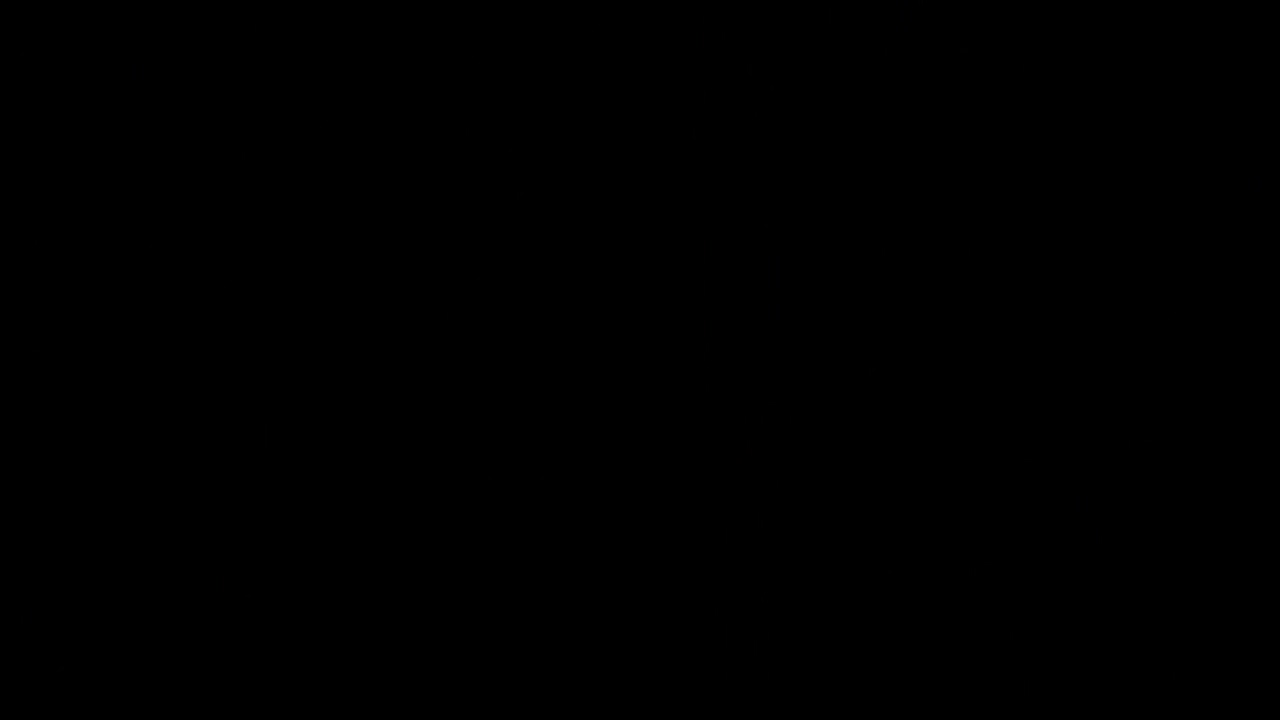The image is a horizontally aligned vertical rectangle filled completely with a solid black color. The blackness is uniform, with no visible text, pictures, shades, highlights, or shadowing. The dimensions appear to be approximately six to seven inches in length and about four to four and a half inches in height. This graphic seems entirely devoid of any light information, making it impossible to discern any details or variations in color. Whether it's a photo of a pitch-dark space, like a night sky or a dark room, or simply an image colored solid black in a paint program, no visual elements are detectable even with maximum screen brightness. It's an image dominated by an absolute, uninterrupted black.